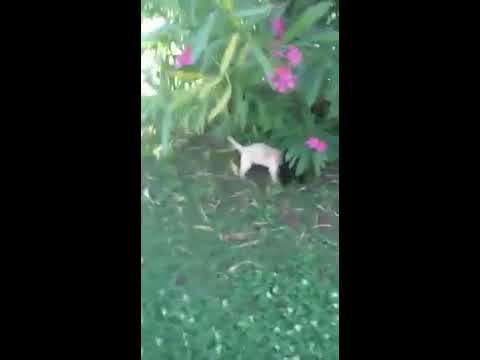In this photograph, taken during the daytime in an outdoor garden area, the ground is covered with green grass, interspersed with patches of brown soil. The focus of the image is a small, somewhat blurry animal, possibly a cat or a small dog, with cream-colored fur. The animal's head is obscured by the leaves of a nearby bush, which is adorned with green leaves and pink flowers. The animal’s erect tail suggests alertness. The scene appears slightly cluttered, as the grass in the foreground looks either freshly cut and not yet raked or littered with fallen leaves. The garden is framed by two vertical black strips on either side, hinting at a possible fence or garden structure. The vertical orientation and overall blur suggest the photo was likely taken with a low-quality cell phone camera.